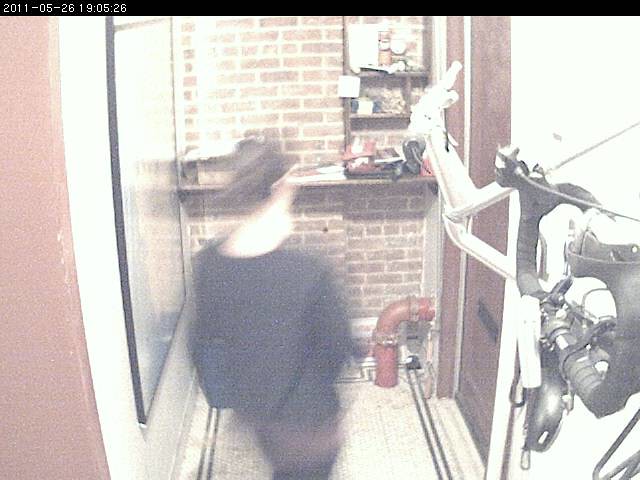The image, likely captured by a low-quality security camera, shows a small, dimly lit room or hallway. The photograph, marked with the timestamp "2011-05-26 19:05:26" at the top, features a blurry figure wearing a black hat and dark clothing walking towards a brown door situated on the right side. The room has a brick wall at the center, adorned with a shelf that appears to hold some tools. A red pipe runs vertically from the ground on the right side. To the left, a white wall displays a painting in a black frame. The image also includes a cabinet full of miscellaneous items, a small brown wall, and what appear to be the black and white handlebars of a bicycle in the bottom right corner. The overall quality is compromised by blurriness and graininess, typical of security footage.